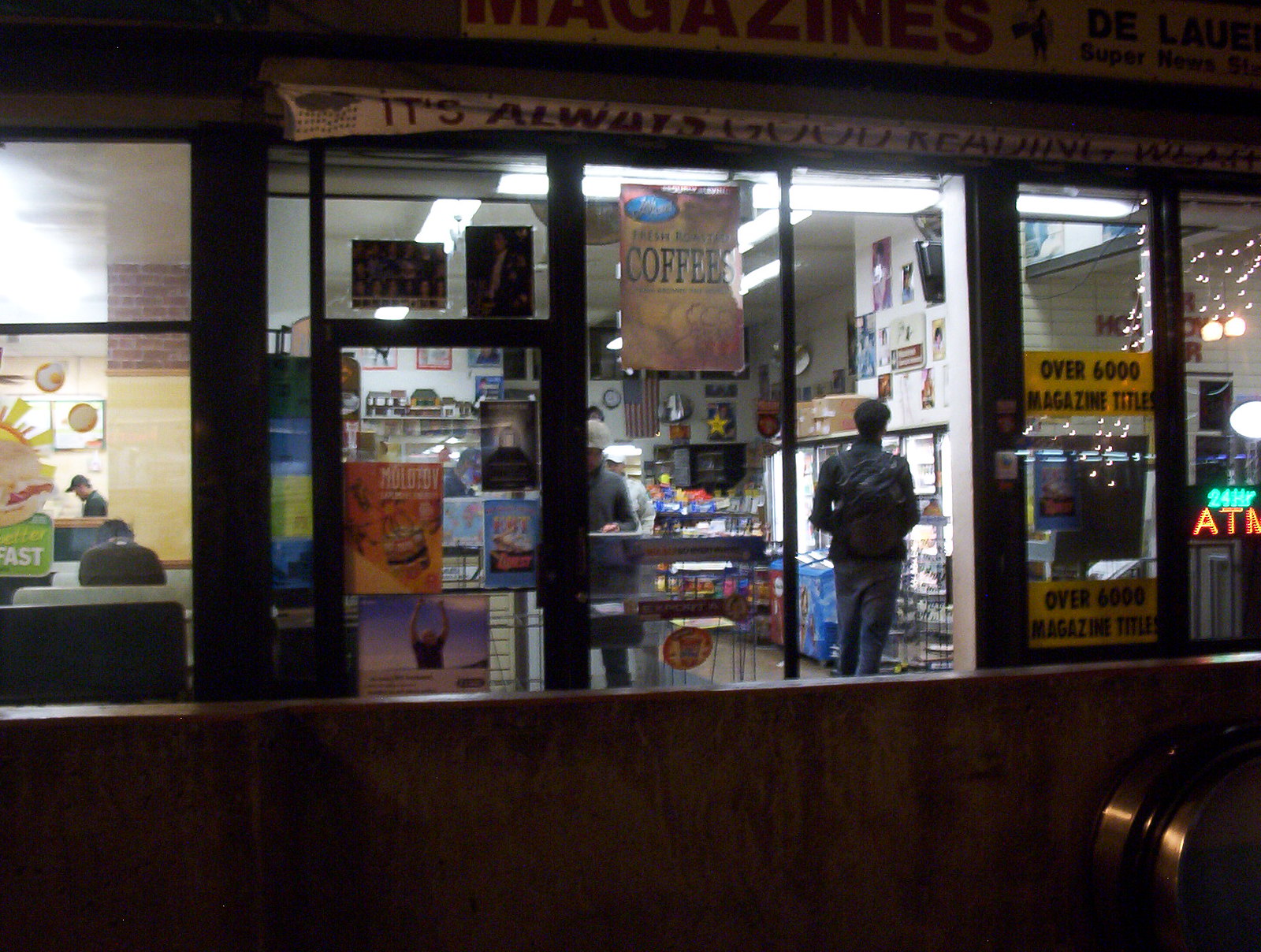The image captures a vibrant urban scene centered around a variety store with a distinct storefront sign reading "magazines" prominently displayed at the top. The photo appears to be taken from the top of an escalator, with the edge of the escalator and a cement wall visible to the right. Below, on the left, is part of a wooden door featuring a golden knob. Adjacent to the variety store on the left is a food shop, likely a Subway, given the recognizable sandwich sign and the word "breakfast" visible on its door.

The "magazines" store itself is well-lit and bustling with activity. Through its large windows and glass door, various advertisements and signs can be seen, albeit some are blurry. Notable signs include one that reads, "over 6,000 magazine titles" and another prominent brown-colored sign reading "coffee." Inside, a man in a black leather jacket and blue jeans draws attention as he looks towards the store's back. Additionally, another customer in a gray shirt and white hat appears to be exiting the store. The interior is adorned with old French tin signs and features an American flag hanging by the register located at the back right of the store. Highlighted by an ATM sign, the variety store seems to offer a wide range of goods from magazines and coffee to likely cigarettes and more.